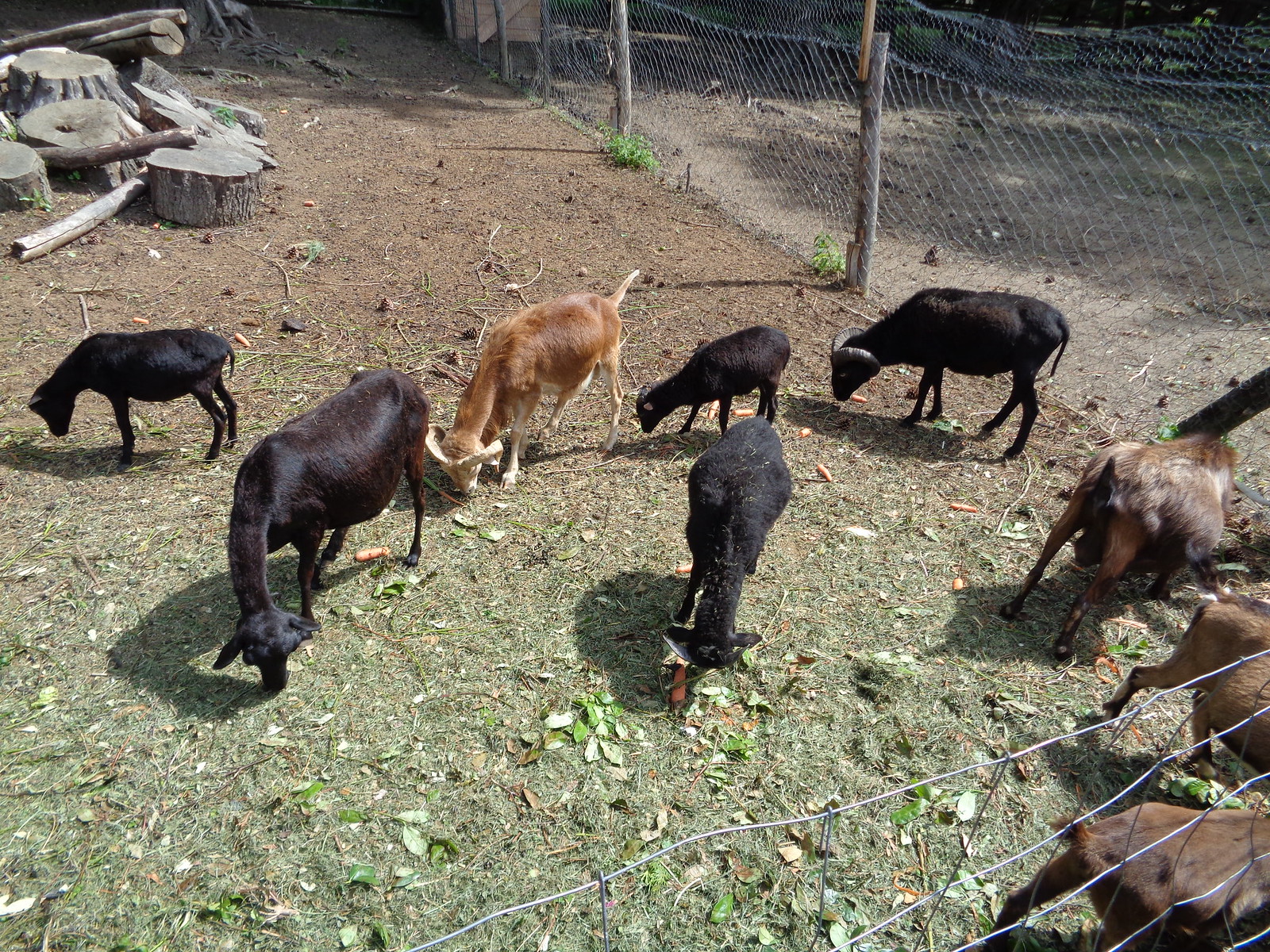The photograph captures a lively and diverse goat pen set within a fenced area that appears to be part of a professionally maintained petting zoo or a farm. The enclosure is defined by a wire mesh fence supported by round vertical wooden posts. Inside the pen, the ground is mostly bare dirt with a scattering of short grass clippings. Several goats are present, displaying a variety of colors and features: there are black, brown, and tan goats, some sporting distinctive horns. A particularly notable goat is a brown one with a lighter colored tail and ears. More reddish-brown goats are visible to the right side of the image, one of which might be a milking goat. None of the goats are looking directly at the camera; instead, they seem to be casually milling about. Visible in the background are several light-gray and brown tree stumps, arranged strategically to allow the goats to jump and play. These stumps and logs contribute to the well-organized, interactive environment, hinting at the care taken to create a stimulating habitat for the goats.